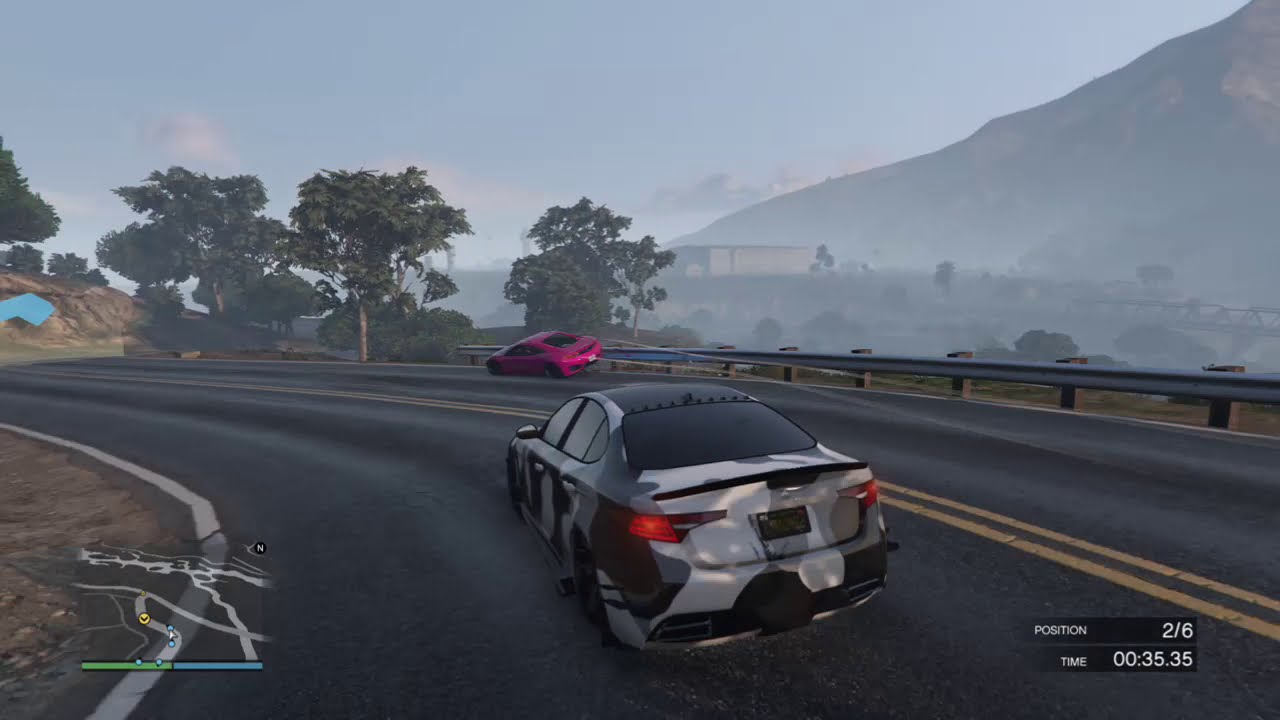This screenshot from the video game "Grand Theft Auto" (GTA) captures an intense moment in a high-speed race. Two high-performance cars, including the player's black Lampadati Komoda with a white camouflage pattern, are rounding a bend on a two-lane mountain road. The car in the foreground is shown from an elevated third-person perspective, about four or five feet away from the camera. Ahead, a red sports car, precariously up on the guardrail, threatens to collide with nearby trees. The asphalt road, marked by a double yellow line, is flanked by guardrails and bordered by a foggy, hazy landscape of mountains and a tree line. In the lower left corner, a mini-map indicates the track layout and the car's position. The bottom right corner displays race information, showing the player in "position 2/6" with a race time of "00:35.35." The backdrop features a blue sky adorned with clouds, enhancing the tension of this competitive scene.